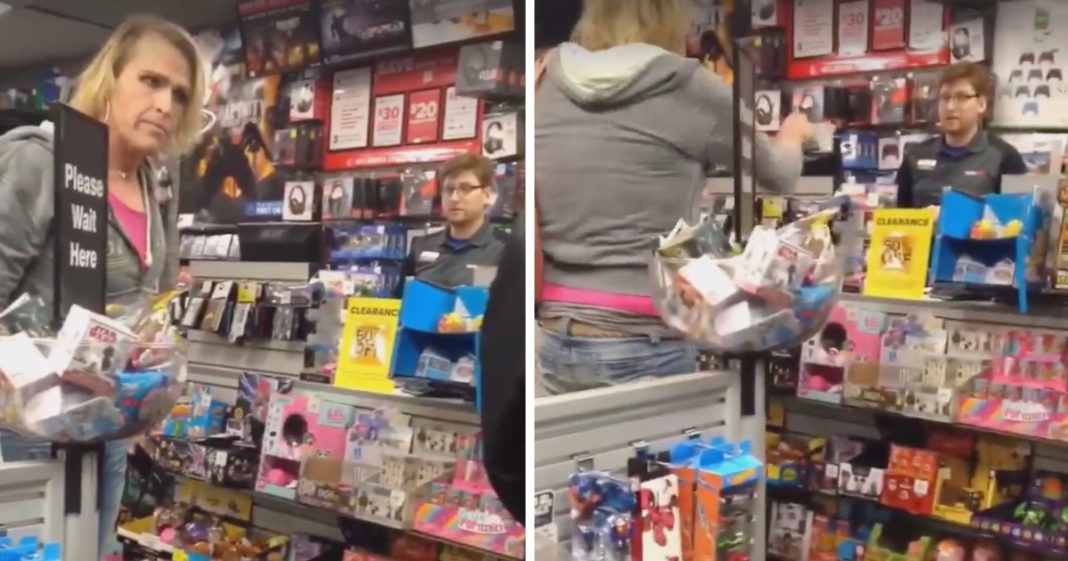The image comprises two side-by-side photos taken inside what appears to be an electronics or gaming store. Both photos showcase a woman wearing a gray pullover, jeans, and a pink shirt standing in line at the counter. In the first photo, she faces the camera while a bearded clerk with glasses, wearing a black shirt and name tag, attends to her. The cluttered counter displays various items, including a yellow sign and a prominent blue rack, with several products such as gift cards (marked $20 and $30), a box of headphones, and other electronics for sale. The background includes a "clearance" sign and boxes with "Star Wars" imagery.

In the second photo, taken from a slightly different angle, the woman has turned towards the clerk, raising her arm as if in conversation, while the clerk looks back at her. The surroundings, including the racks and signage, are consistent with the first image, reinforcing the impression of a store specializing in electronics or gaming merchandise. Despite the slightly blurred quality of the images, the scene vividly captures the typical layout and atmosphere of such retail environments.